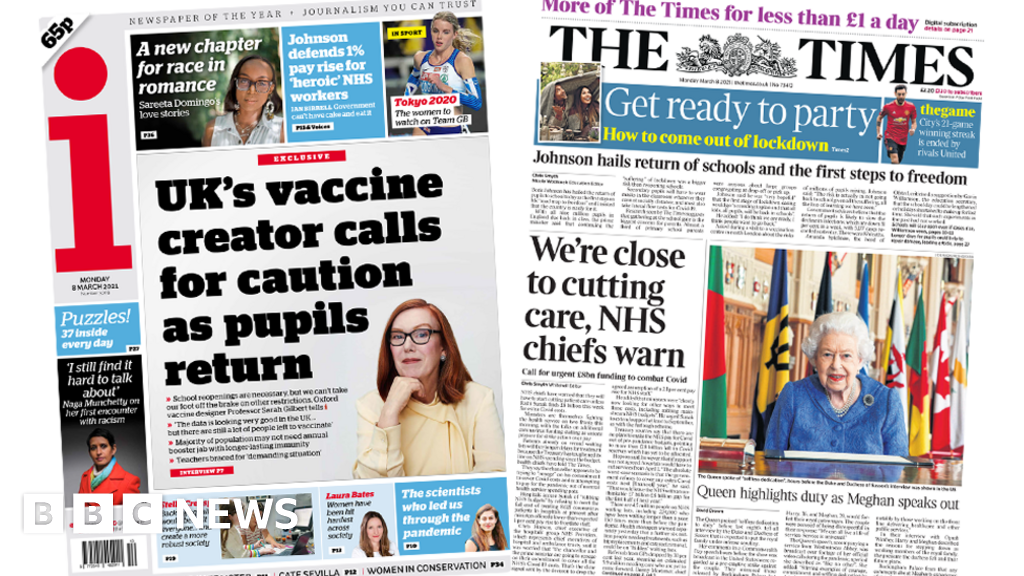Photograph of Two UK Newspapers – The image depicts two UK newspapers placed at slight angles to each other; the newspaper on the left is tilted slightly to the left, and the one on the right is angled a little to the right. The left newspaper is priced at 65p, labeled with a capital "I" proclaiming "Newspaper of the Year" and "Journalism You Can Trust." This is an actual physical newspaper as evidenced by the barcode and price at the bottom.

The main section of the left newspaper features three prominent images at the top. Headlines include "A New Chapter for Race and Women," "Johnson Defends 1% Pay Raise for Heroic NHS Workers" in the center panel, and "Tokyo 2020" showcasing a blonde-haired runner. The central highlight is "UK's Vaccine Creator Calls for Caution as Pupils Return," accompanied by various other options and articles at the bottom.

The right newspaper, identified as "The Times," announces "Get Ready to Party, Had to Come Out of Lockdown" as its focal headline. Other significant headlines include "We're Close to Cutting Care—NHS Chief Warns," and "Queen Highlights Duty as Meghan Speaks Out," juxtaposed with her image. At the top, it reads "Johnson Hails Return to Schools in the First Step to Freedom," and there’s also a runner pictured to the right under the main logo. A portrait of the Queen features prominently, emphasizing her continuing role, underscored with extensive text.